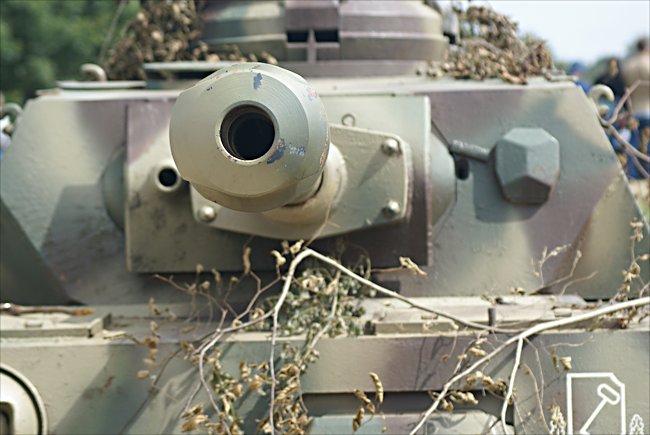The image captures the front side of a large, silver-toned armored tank, likely set in a woodland area. The central focus is the barrel of the tank that projects outward, adorned with a distinctive donut-shaped ring at its tip. This barrel extends into the rectangular "head" of the tank, which features intricate geometric patterns, including diamond-like designs and a hexagon shape to its right. Entangled with dead and dried branches and leaves, the tank appears camouflaged, suggesting it has either maneuvered through dense foliage or been deliberately disguised. The body of the tank is relatively slender and includes a logo resembling an SD card on the lower right-hand side. A blurred forest backdrop enhances the scene with out-of-focus trees, and three people in blue, black, and taupe jackets can be discerned in the background to the right, hinting that the setting might be part of a historical reenactment or outdoor exhibit.